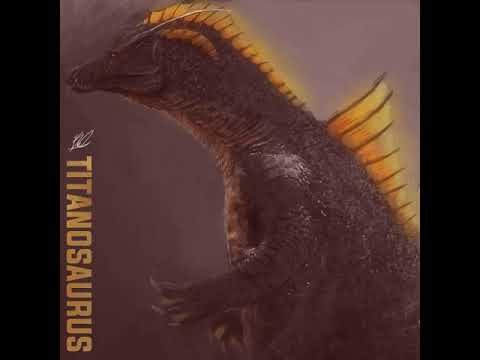The image is a detailed, colored illustration of a dinosaur labeled "Titanosaurus," depicted in a side profile view. The background features a brown and black gradient with two black stripes on either side. The dinosaur, primarily yellow and orange with rough-textured scales, has a pointy, wolf-like head with a pronounced snout and small ears. Its body is adorned with spines or fins running down from the top of its head to its back. Only the dinosaur's upper body is visible, showing three-fingered claws or hands. The dinosaur is positioned more towards the right, seemingly walking on two legs, although its lower legs are not visible. The word "Titanosaurus" appears in yellow capital letters, slanted and positioned along the left side of the image. The overall aesthetic suggests a science-based context, akin to a magazine cover or a CD featuring dinosaur imagery.